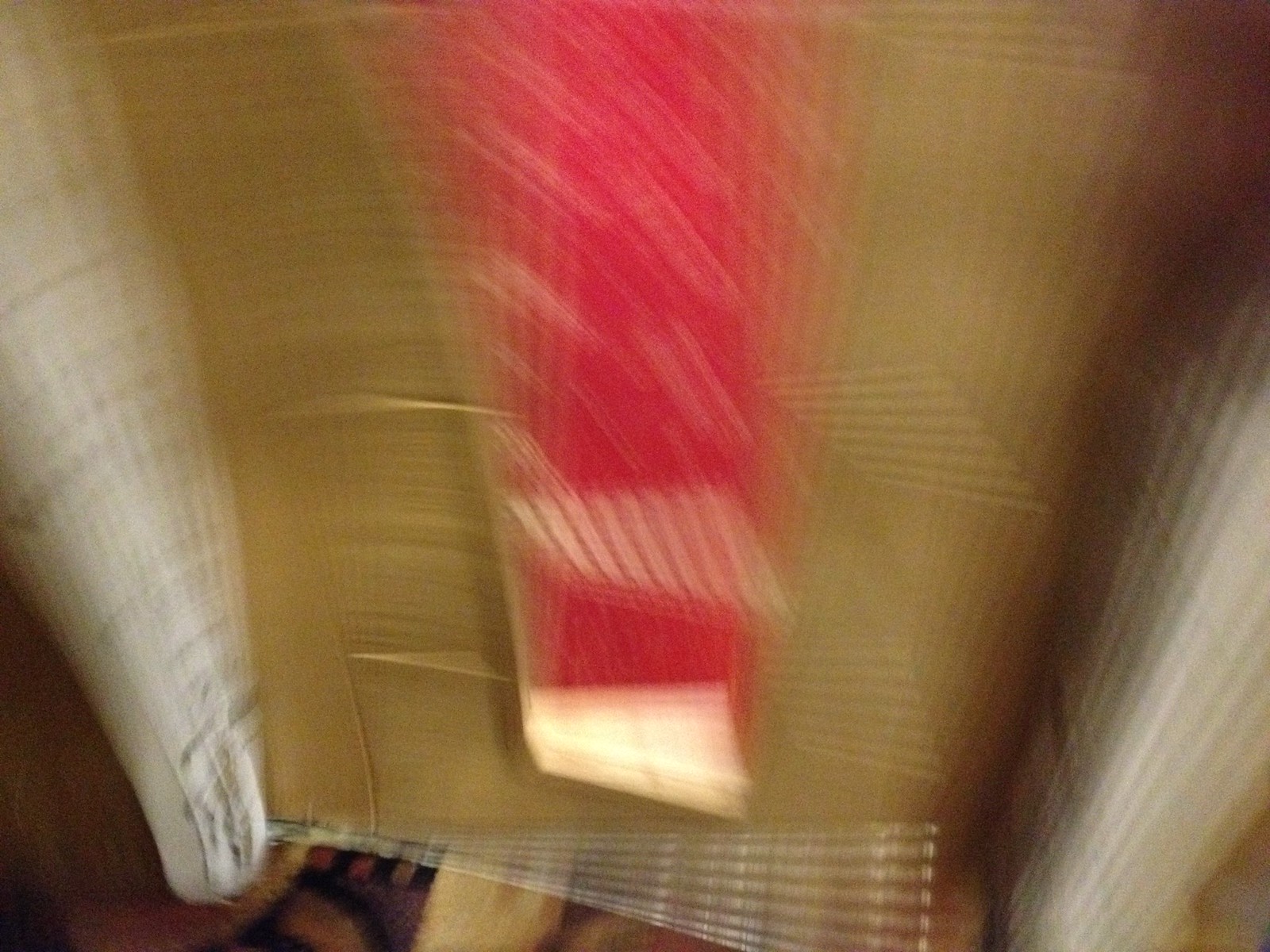This close-up photograph is heavily blurred and difficult to identify, evoking a sense of motion. At its center, there's a red section flanked by golden-brown shapes that form a rough U shape. These shapes are bordered by white objects on both the left and right sides. The foreground contains a patterned carpet or similar texture, adding to the complexity. The image's blurriness exaggerates repetitive lines and streaks, giving an illusion of continuous movement whether you focus directly on it or glance around. It could be a cardboard box with cutouts revealing an interior, or it might depict the back of a chair with some fabric, such as a pink scarf, draped over it. The exact subject is ambiguous due to the intense blur and close proximity of the camera.